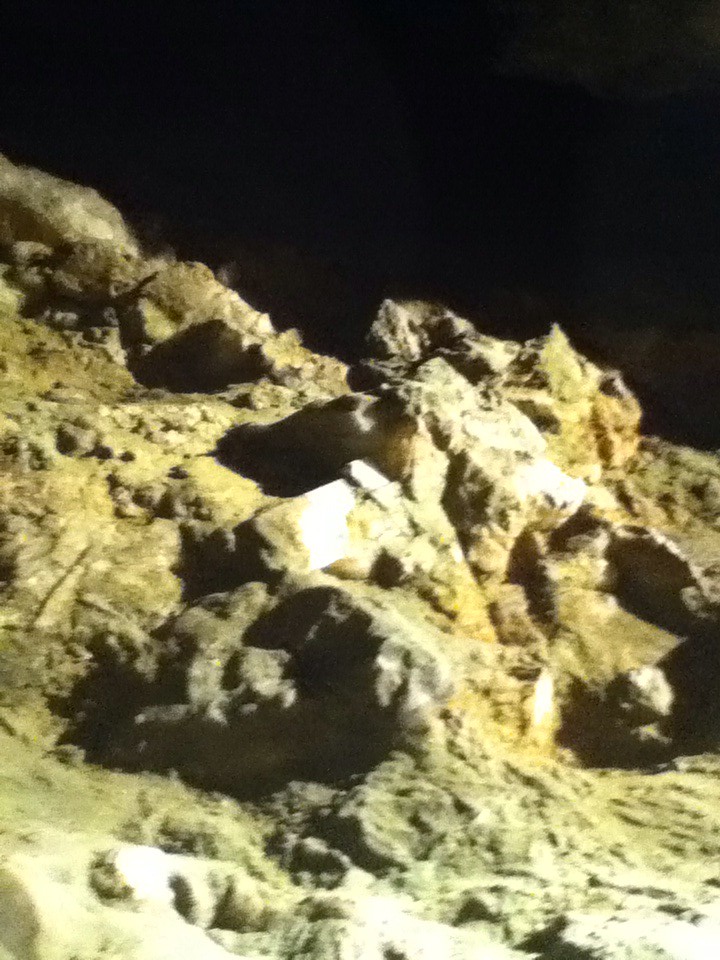This vertically aligned photograph depicts an outdoor rocky formation during the day. The top third of the image is a solid, pitch-black backdrop that contrasts sharply with the illuminated rock formation below. The rocky surface begins in the upper left corner and slopes downward to the middle right section, displaying a varied and uneven texture. In the upper left, the rocks appear darker brown, transitioning to lighter brown and tan as the slope progresses downward. The central section showcases the largest chunks of rock, which include mixes of gray, white, and orange or golden hues, likely highlighted by sunlight casting shadows on certain parts. The foreground features distinct gray rocks and a prominent white rock, adding to the textural complexity of the scene. The photograph captures a rugged, sunlit terrain with a dynamic play of light and shadow, set against a stark black sky, emphasizing the raw, natural beauty of the rocky landscape.